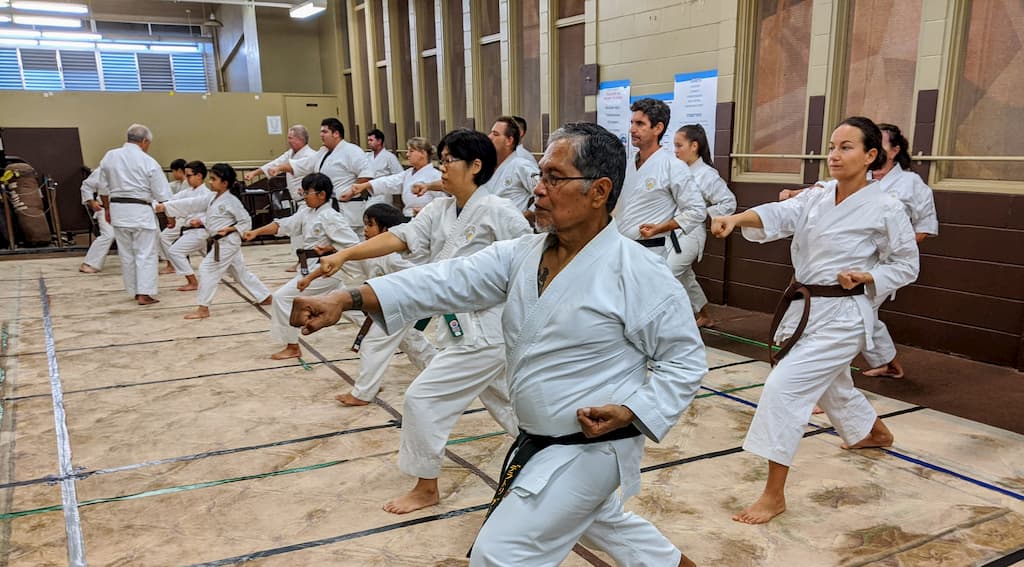This image depicts a diverse martial arts class set in what appears to be a community center. The group includes men, women, and children, all dressed in traditional white martial arts uniforms with belts around their waists, indicating varying levels of proficiency. The scene captures a moment where all participants, positioned in three rows, are executing a synchronized move: their right fists are extended forward, their left fists are held by their sides, with one leg forward and the other slightly bent back, forming an 'A' shape with their legs. The instructor, an older gentleman with gray hair, can be seen moving through the rows, providing corrections and encouragement.

The class is conducted on a floor with a pattern of gray taping or rectangular shapes, adding to the structured environment. The backdrop features a mix of dark brown bricks at the bottom and tan or light brown bricks extending upwards, complemented by numerous windows that allow natural light to stream in. In the far left corner, you can glimpse a piece of exercise equipment, adding to the impression of a multi-functional community space. The overall atmosphere seems lively and disciplined, with the instructor's presence ensuring a focused practice session.